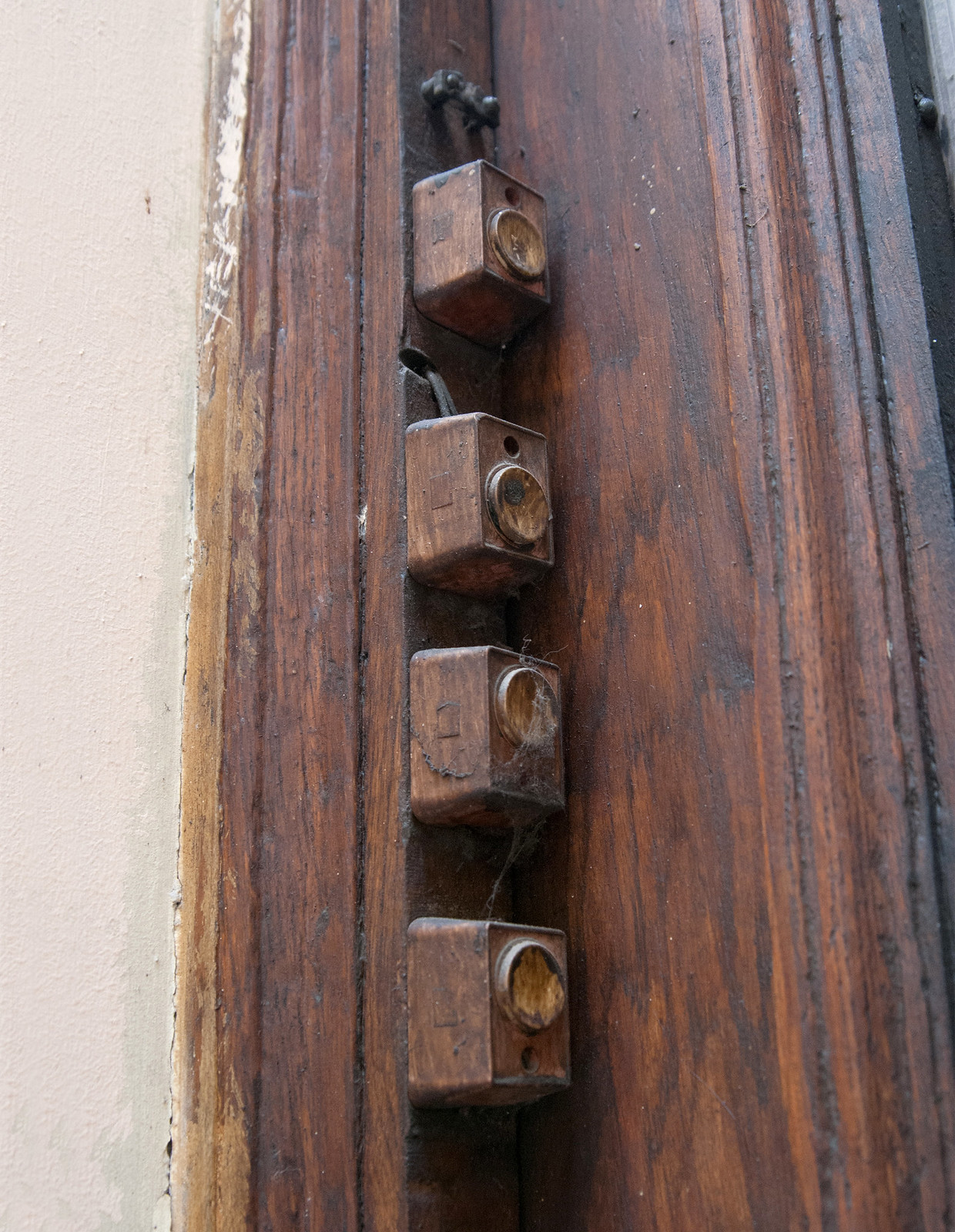This is a close-up, portrait-style image of a weathered, old wooden doorframe connected to a wall, likely at the entrance of a building. The wood is rough and dirty, adorned with cobwebs and spots of peeling paint. On the left side of the image, there's a partially painted white wall. Prominently featured on the wooden frame are four small, box-like, orange electrical units, each resembling the size of ring boxes, and they are aligned vertically. These boxes are interconnected with black electrical cords. Cobwebs cover the boxes, and each has a small circular disc on top. The uppermost box has two black screws above it. Due to their positioning and appearance, these boxes might function as doorbells for individual flats or businesses, allowing visitors to press them to gain attention inside.